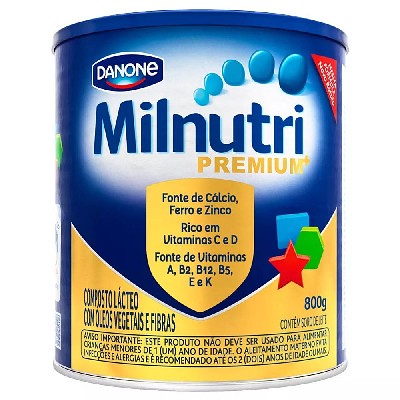The image features a can from the brand Danone, prominently displayed against a solid white background, giving it a cut-out appearance. The can, primarily colored in blue, white, and gold with touches of red, is labeled "Milnutri Premium." The brand logo, "Danone," is situated in the top left corner within a blue, squared-off oval, featuring white lettering and a subtle smile curve in light blue and red underneath.

The central design of the can includes the text "Milnutri" in dark blue, transitioning to "Premium" written in a golden-yellow color. Just below "Premium," there's a gold, shield-shaped silhouette containing additional dark blue text in another language. Above this is a collection of elements including blue circular shapes, a slight red downward-pointing triangle banner, a red star, a green octagon, and a blue square—all adding visual interest. At the bottom right of the can, "800 grams" is clearly marked in blue text.

The lower portion of the can is primarily gold-yellow, complementing the premium branding, and a paragraph of descriptive text in another language is also visible here, contributing further detail to the product's packaging.